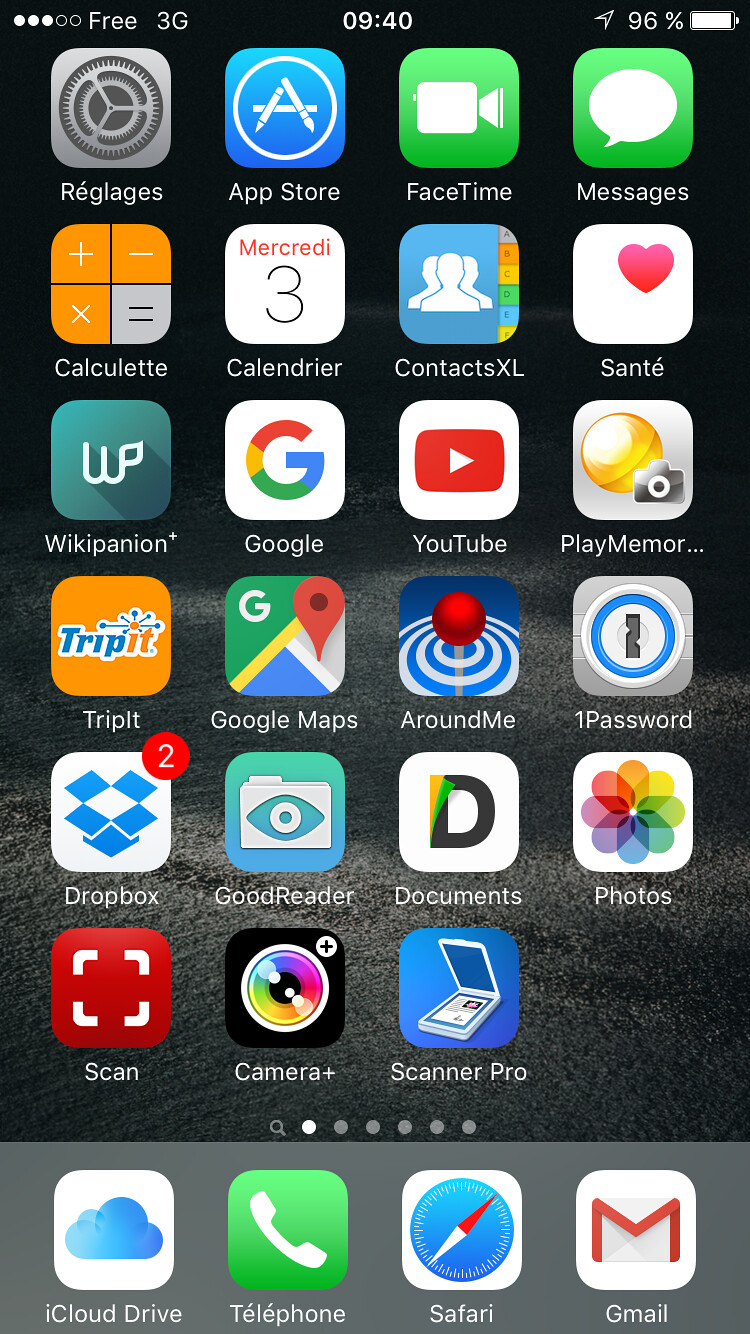This is a detailed caption of a smartphone screenshot showcasing a cluttered home screen filled with various apps. The digital clock at the top center displays the time in military format, reading 0940. The top left corner features small white text indicating "free," while the status bar to the right shows a 3G network connection. On the top right, a paper airplane icon is present next to a 96% battery indicator, suggesting a nearly full charge.

The home screen is densely packed with apps, leaving only a small empty space in the bottom right corner. The apps do not appear to follow any particular order. Notably, the top left app is labeled "Rigogulous," and just below it, another app is named "Calculate." These names indicate that the smartphone likely belongs to a non-English speaker. Among the more recognizable English-named apps are Dropbox, Documents, and Photos.

At the bottom of the screen, four staple apps are anchored: iCloud Drive, Telephone (an app for making calls, labeled with the word "Telephone"), Safari (the browser), and Gmail. The variety of apps and their disorganized placement give insight into an extensive and varied app usage by the phone's owner.